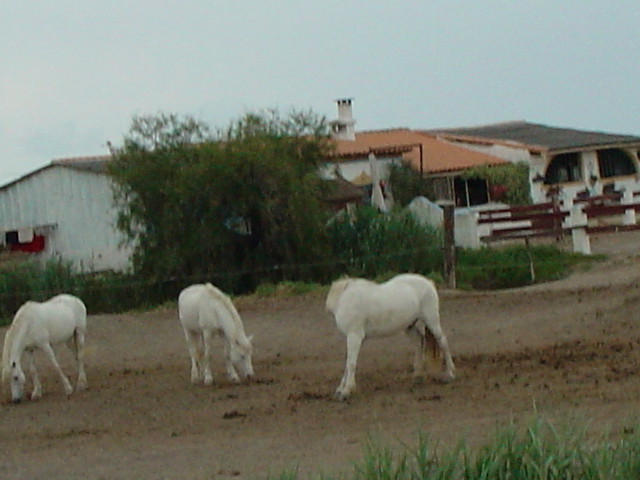This outdoor daytime photograph captures a serene scene under a dark, cloudy sky. The focal point is three small, white horses or ponies grazing in a dirt area. Two of the horses have their noses down to the ground, seemingly searching for food, while the third horse turns its head to the side, possibly to scratch an itch. In the lower right corner, there's a patch of grass contrasting with the dirt they're grazing on.

In the background, there is a series of white buildings, including a single-floor house that appears wooden with a mixture of red-brown and white walls. The house features a chimney in the center and is surrounded by a wooden and wire fence. The left side of the house is partially obscured by tall bushes or short trees, while the right side is accompanied by what looks like a stable with two open, glassless windows and a gray roof. A smaller building to the far right also forms part of the backdrop, potentially serving as a barn, given its proximity to the horses. The roofs of the buildings vary in color, with one being black, another red, and the color of the far-left building's roof being indiscernible. This photograph, though faded and poorly lit, captures a peaceful rural tableau.